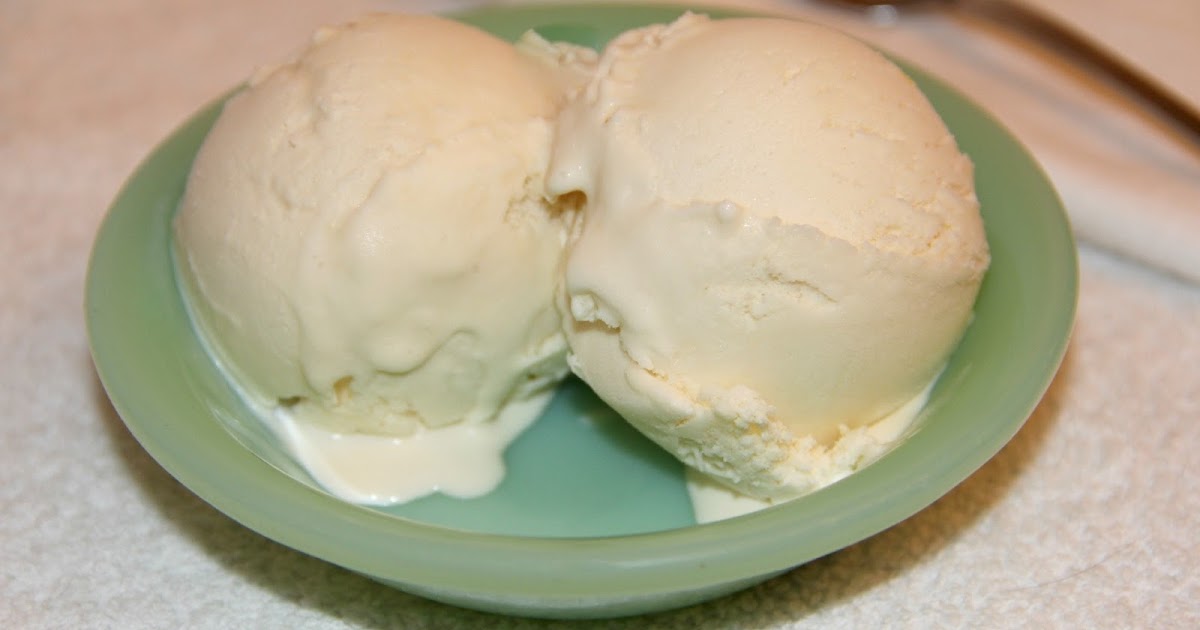This color photograph, in landscape orientation, captures a beautifully detailed scene of two slightly melting spherical scoops of vanilla ice cream, nestled together in a pastel green, round dish. The scoops, almost leaning against each other in the center of the dish, create small puddles of cream-colored liquid at the bottom. The dish, which evokes a vintage 1950s or 60s aesthetic, sits atop a creamy white tablecloth. The tablecloth, beneath the dish, features dark red and light blue stripes near the top right corner, adding a subtle hint of color to the otherwise serene palette. In the background, some silverware peeks out from the right-hand side, suggesting this setting might be a traditional kitchen table. The photograph is well-lit with natural indoor lighting, enhancing the soft, nostalgic feel of the scene.